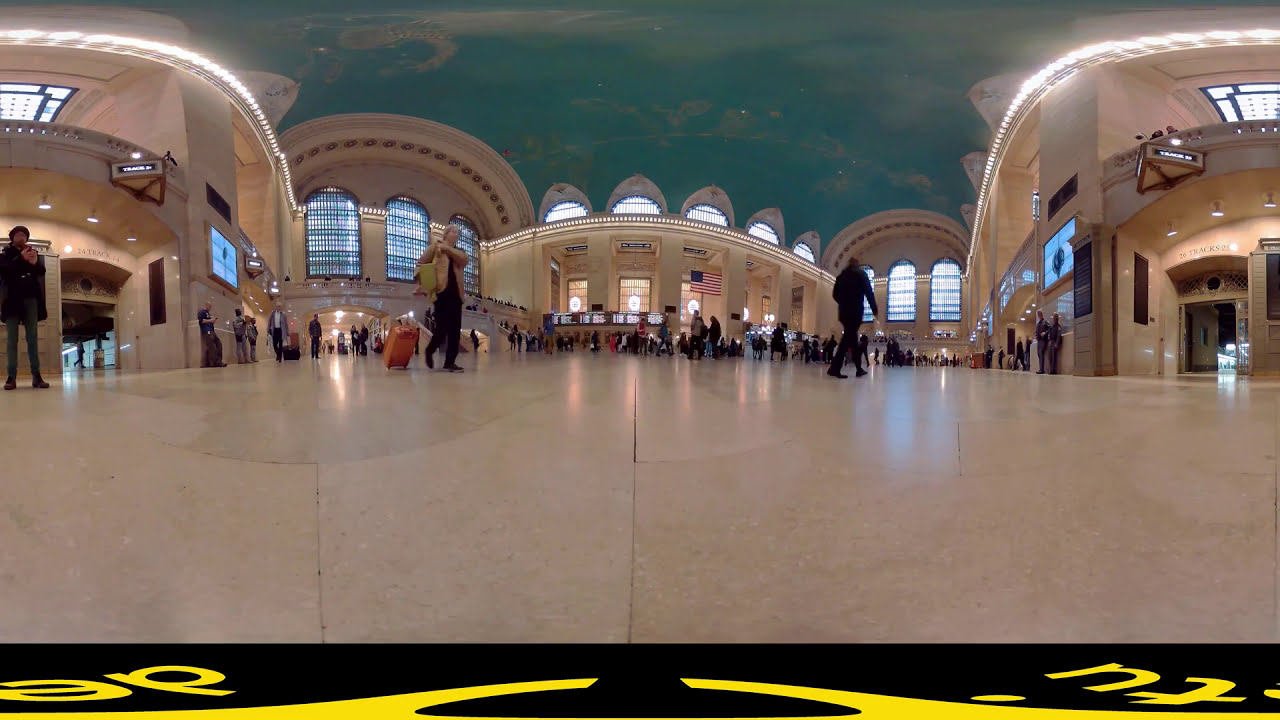This is a slightly warped, low-resolution 360-degree panoramic photograph depicting a bustling train station. The image shows a large room with light brown stone tile flooring and matching stone-colored walls. The ceiling, painted a bright blue with misty white cloud-like designs, gives the impression of a sky. Ornate Roman and Italian architectural features, such as large arches near the ceiling and numerous large windows with multiple panes, adorn the space. Rows of bright electric bulbs line the ceiling, adding to the well-lit ambiance.

In the distance, we see large crowds of people, some dragging bags or carry-ons, indicating an active travel hub. An American flag and various signs, including electric and regular screens, are visible on the far wall along with some notice boards and display monitors. There are intricate entrances and exits, an upper deck accessed by a staircase, and several alcoves and doorways throughout the area. The smooth marble-like floor enhances the room's elegance, while assorted video monitors and bright lights contribute to the vibrant atmosphere. In the foreground, a person with an orange suitcase stands out, emphasizing the travel-centric nature of this grand, vintage-style station.